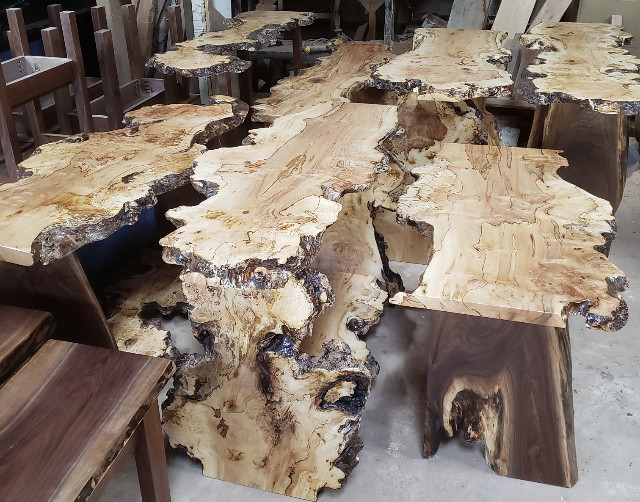The image depicts a detailed and well-crafted display of wooden furniture within a wood shop, set against a concrete floor. Central to the scene are six to seven unique tables, meticulously fashioned from natural tree trunks. Each table showcases a flat top surface, reflecting a light tan hue with darker brown accents, and they are elevated by natural wood bases that retain their organic shape, echoing the tree's original growth pattern. The sides of these tables, depicted as polished rich brown, beautifully contrast their lighter tops. 

Additionally, the woodwork reveals intricate, irregular carvings that lend an authentic, jagged edge to the pieces, with some tables displaying noteworthy knots and textures. Behind these tables, partially visible, are other wooden items including chairs—some of which appear flipped with their legs pointing up—and smaller benches or tables. The background includes a variety of wooden panels and further furniture items in various states of assembly or display, underscoring the artisanal nature of the wood shop setting.